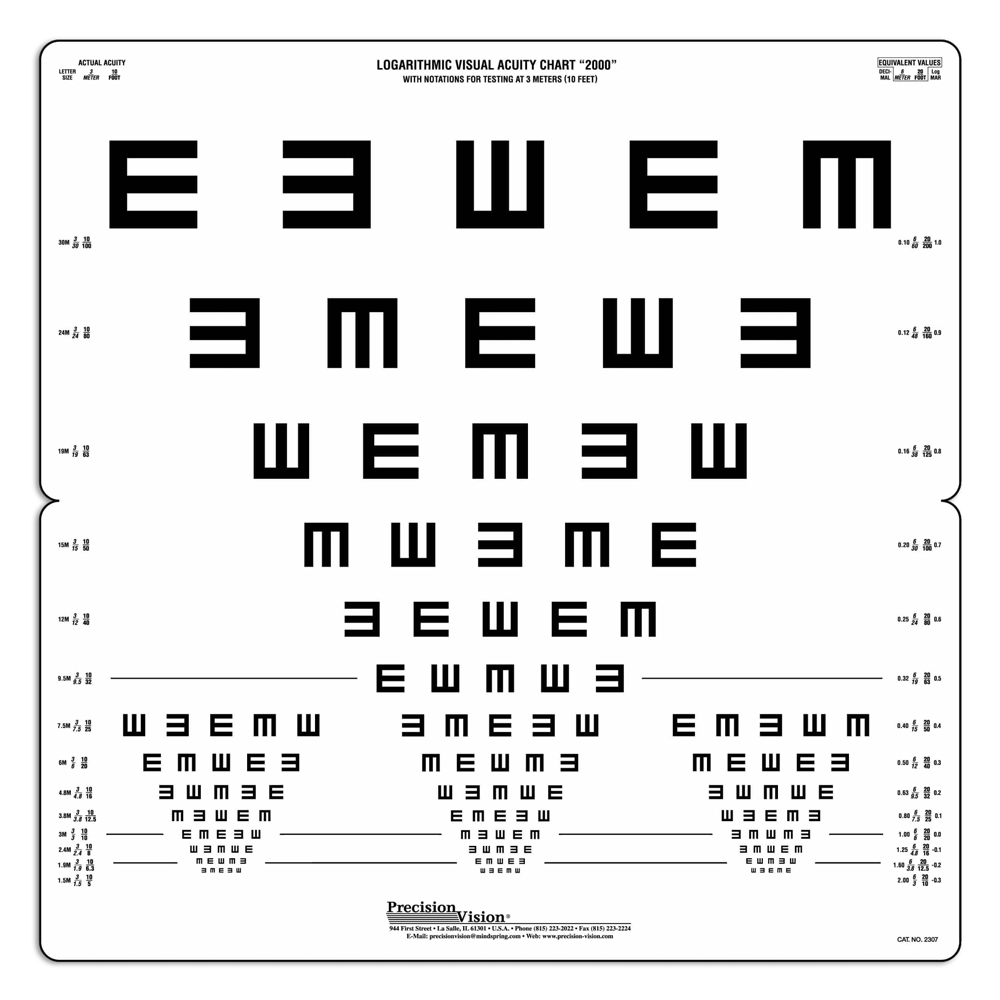The image depicts a logarithmic visual acuity chart commonly used by optometrists to measure a person's visual distance and clarity. At the very top of the chart, small black text reads "logarithmic visual acuity chart, 2000" with notations for testing at 3 meters (10 feet). The chart features the letter "E" in various orientations, such as standard (facing right), reversed (facing left), upside down (pointing downward and resembling an "M"), and pointing upwards. The letters are arranged in rows, starting with larger symbols at the top and progressively smaller ones towards the bottom, creating a funnel-shaped pattern that challenges visual acuity as it reduces in size. Notably, "Precision Vision in LaSalle, Illinois" is indicated on the chart. Additionally, there are two smaller funnel-shaped diagrams on the bottom left and bottom right of the main chart for further detailed assessments.